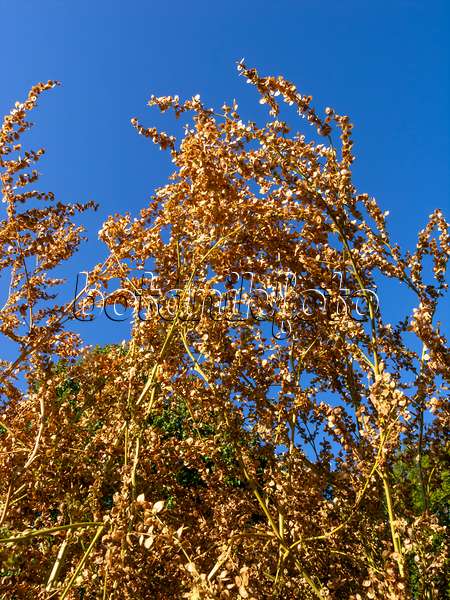The photograph captures a striking scene of a tall, twisted bramble of branches and dead, tall weeds set against a vibrant blue sky. The seemingly lifeless bush, with its tangle of thin, sharp, and possibly prickly branches, displays an array of dried leaves and small petals in shades of brown, orange, and gold. The branches and leaves appear rough and dry, suggesting the plant's possible demise. Sunlight illuminates the front of the bramble, emphasizing the stark contrast between the dead branches and the deep blue sky. In the background, a glimpse of greenery, possibly bushes or trees, adds a touch of vibrant life to the scene. A transparent watermark at the center, reading "Botanaphoto," subtly marks the image.